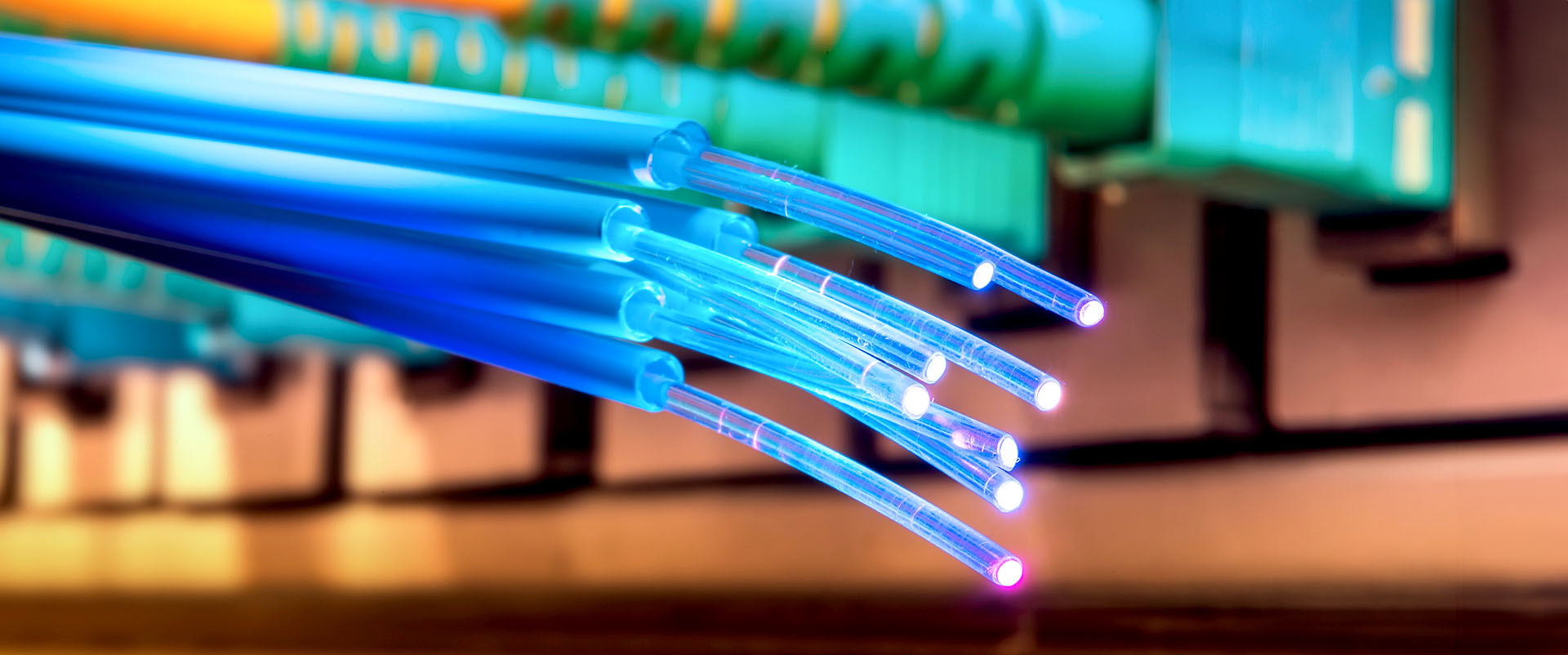The image is a full-color, indoor photograph featuring a high-tech scene dominated by several neon blue fiber optic cables. These cables, numbering around eight, originating from the upper left corner, arc towards the center of the frame. Each cable splits into smaller, straw-like tubes that emit glowing lights, primarily blue but also tinged with hints of purple. The tips of these smaller tubes are brightly illuminated, suggesting active fiber optics. The background is blurred, but faint impressions of teal blue and orange hues are visible in the upper left section, perhaps from other wires or plugs. The lower portion of the background exhibits a mix of beige and black tones. The setting appears to be highly technical with electronic components shrouded in an almost ethereal glow, but the exact nature of the devices is indiscernible. The backdrop is white with a blurry texture, bordered in black.